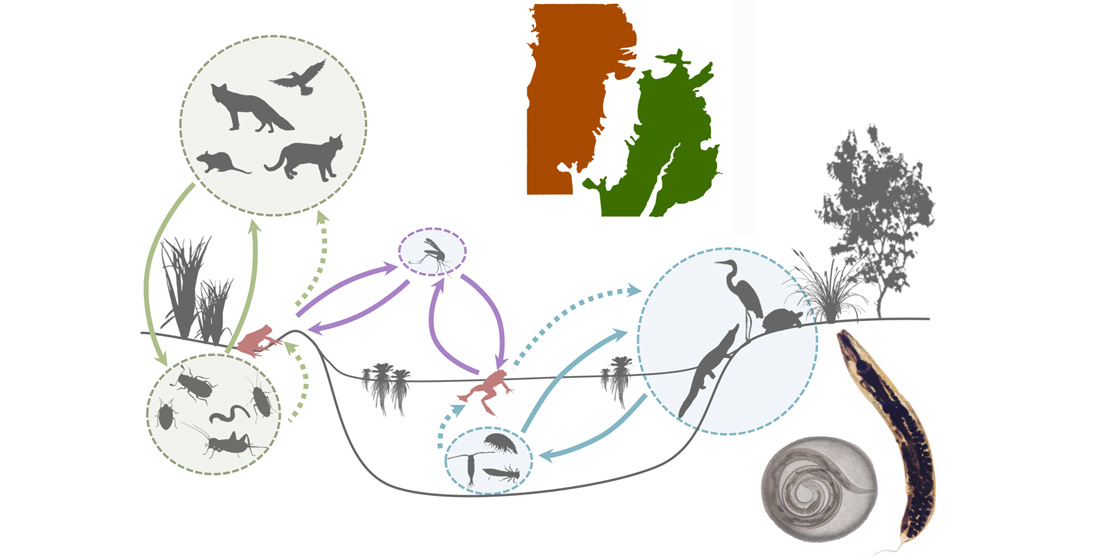This image depicts a detailed ecosystem flowchart. At the top center of the image, two landmasses are depicted in color—one orange on the left and one green on the right. Below these landmasses is a black-and-white section with blue and purple arrows illustrating interactions among various species. 

In the top left corner, a circle includes a wolf, a bird, a rat, and a cat, surrounded by arrows indicating various ecological interactions. Below this, an area of black grass connects to another circle containing various insects, with arrows pointing to and away from it. To the right of the mammals and birds, another circle features a mosquito, with arrows showing its relationship to a nearby frog jumping in a body of water.

Adjacent to the frog, which connects back to the insects through an arrow, there are floating plants. Below the frog, in the water, another set of circles contains three insects with arrows linking them both upwards and downwards. A piece of grass floats between two blue arrows also in this water area. A circle at the water's edge contains animal interactions: a crocodile emerging, a stork standing in front of it, a turtle behind the stork, and a sapling next to the turtle leading to a large tree.

In the color section below these interactions, a black worm-like organism appears. To its left, a circular shape suggests a tapeworm or similar organism. On the right, there are x-ray-like images of various insects and outlined trees, indicating detailed biological elements. Overall, the flowchart illustrates a complex web of interactions among terrestrial and aquatic species, highlighting their interconnected roles within the ecosystem.